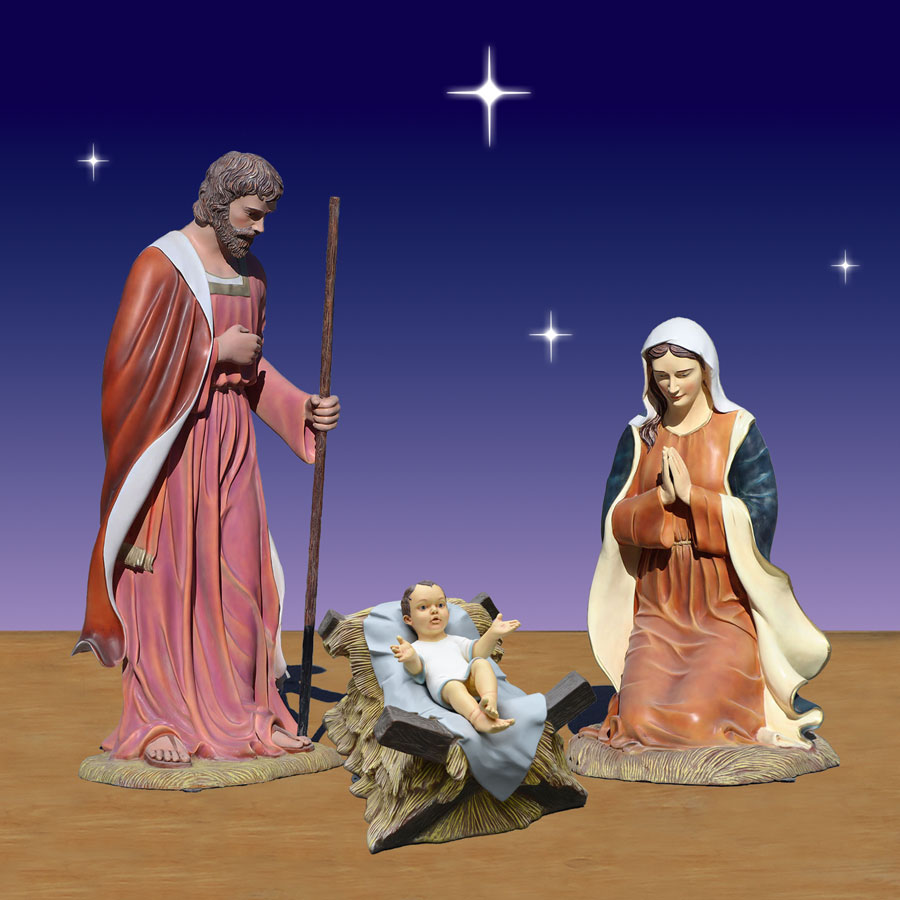This image depicts a classic nativity scene set against a gradient evening sky that transitions from deep dark blue at the top to purple at the bottom, dotted with four twinkling stars, including a partially visible large star at the top. At the center lies baby Jesus in a straw crib, wearing a white robe with blue trim and a baby blue blanket underneath, his tiny arms outstretched. To his right kneels Mother Mary, draped in an orange-red robe, a white veil, and a dark teal cloak with a cream lining, hands clasped in prayer. To the left stands Joseph, clad in long reddish robes and a dark red cloak with a white lining, holding a wooden staff. The scene, rich in color and detail, evokes a traditional Christmas spirit with its ceramic-like figurines positioned on a brown landscape, highlighting the sacred moment.